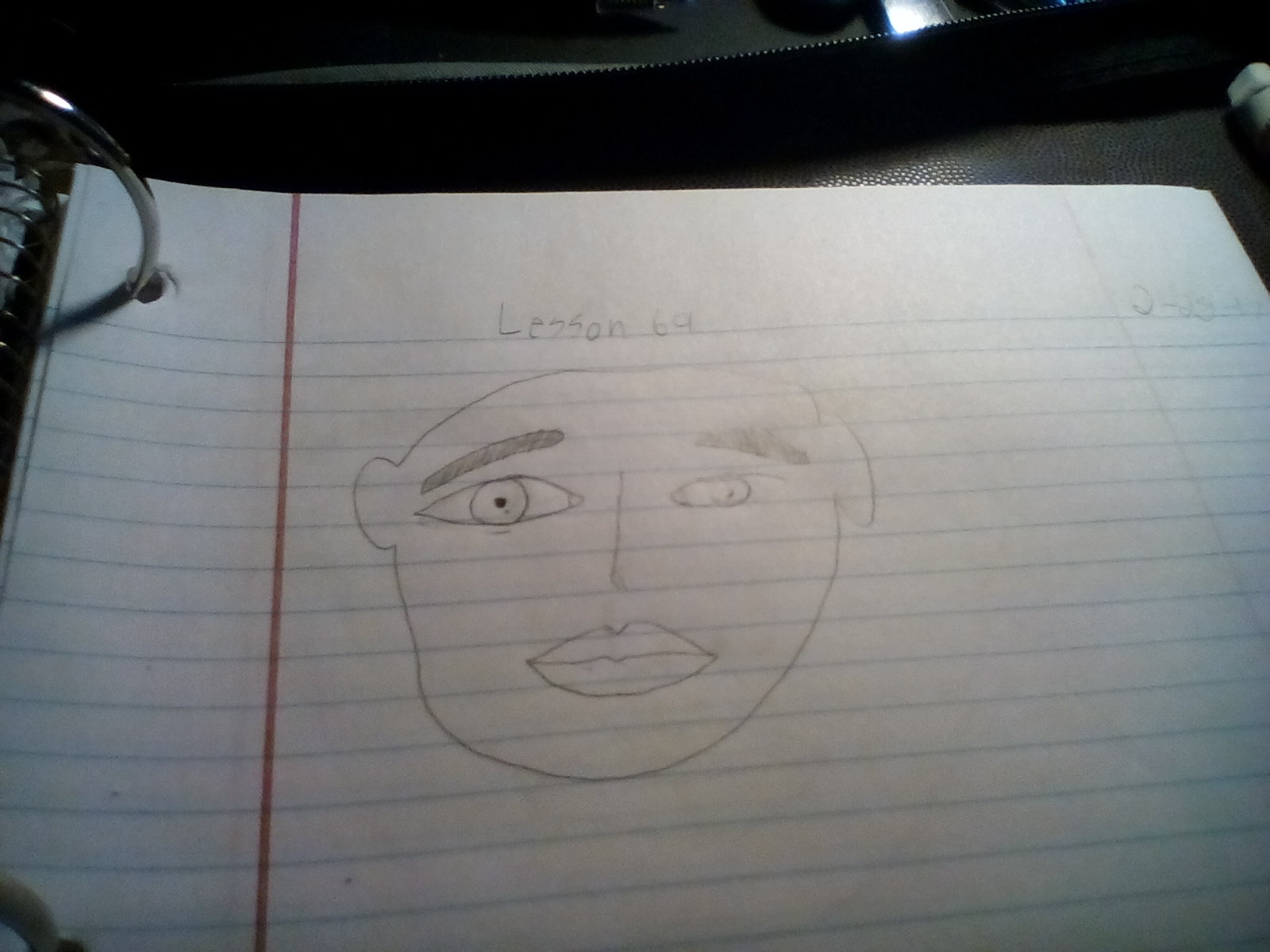This color snapshot reveals a piece of white lined school paper from a large spiral notebook, partially visible within a leather-bound case—the zipper of which is present at the top of the frame. At the top of the paper, written in a somewhat childish hand, is the text "Lesson 69." Below this, a rudimentary, amateurish sketch of a human face is displayed. The face features two asymmetric eyes - the right one being noticeably larger than the unfinished left one. The eyebrows also differ in length, with the right one being longer. The nose is depicted simply with a vertical line resembling an "L" shape. The lips are notably thick, with the left side narrower than the right. The sketch includes a continuous outline tracing the forehead, circular left ear, leaf-shaped right ear positioned higher, cheeks, and chin, but no hair. The details become more evident against the backdrop of the blue horizontal and red vertical lines typical of college-ruled paper, emphasizing the simplicity and beginner nature of the drawing.